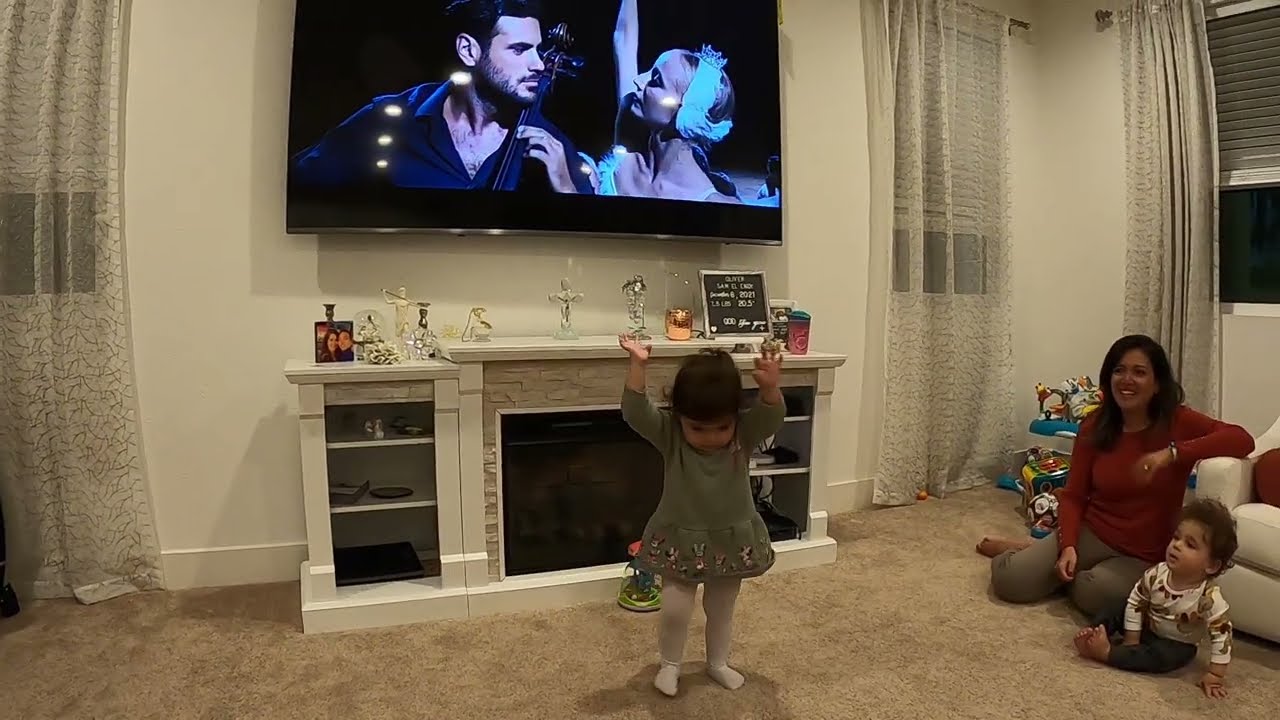The photograph captures a warm, well-lit living room scene featuring three people. To the left stands a little girl, around two years old, dressed in a green dress with embroidered Snoopy designs. She has her hands raised above her head, appearing to dance or imitate a ballerina, mirrored on the large screen TV at the back of the room. The girl has black hair and is also wearing white stockings, standing in front of a white fireplace adorned with knick-knacks. 

Next to her, on the floor, is a younger boy, about 16 months old, dressed in black sweatpants and a white long-sleeved shirt with little designs on it. He sits near a smiling woman, possibly their mother, who is wearing a red sweater and gray pants. The woman is seated on the tan carpet, leaning with her elbow on the arm of a white couch, while looking affectionately at the dancing girl.

The room features white walls, semi-transparent white curtains, and a big screen TV displaying a program with a ballerina and a male dancer, complementing the little girl’s joyful movements. The overall atmosphere is cozy and filled with family warmth and playful interaction.